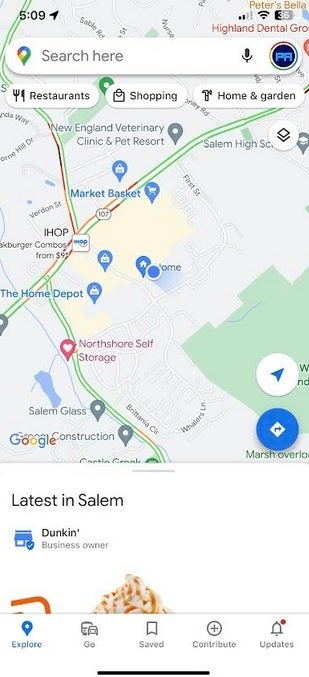The image captured from a smartphone screen displays important on-screen details. In the upper left corner, the time reads 5:09, accompanied by a Wi-Fi signal strength of two bars and a battery life of 36%. Below, the interface features a Google search bar labeled "search here," and includes a black microphone for voice input and a blue circle icon with "PR" inside. Beneath the search bar are three navigational tabs labeled "Restaurant," "Shopping," and "Home and Garden."

Further down the screen, a map is displayed, pinpointing various locations and facilities relevant to a traveler. Key landmarks identified on the map include New England Veterinarian Clinic and Pet Resort, Salem High School, Market Basket, IHOP, The Home Depot, North Shell Self Storage, and Salem Glass. Below the map, a section titled "Latest in Salem" is visible, potentially offering up-to-date local information.